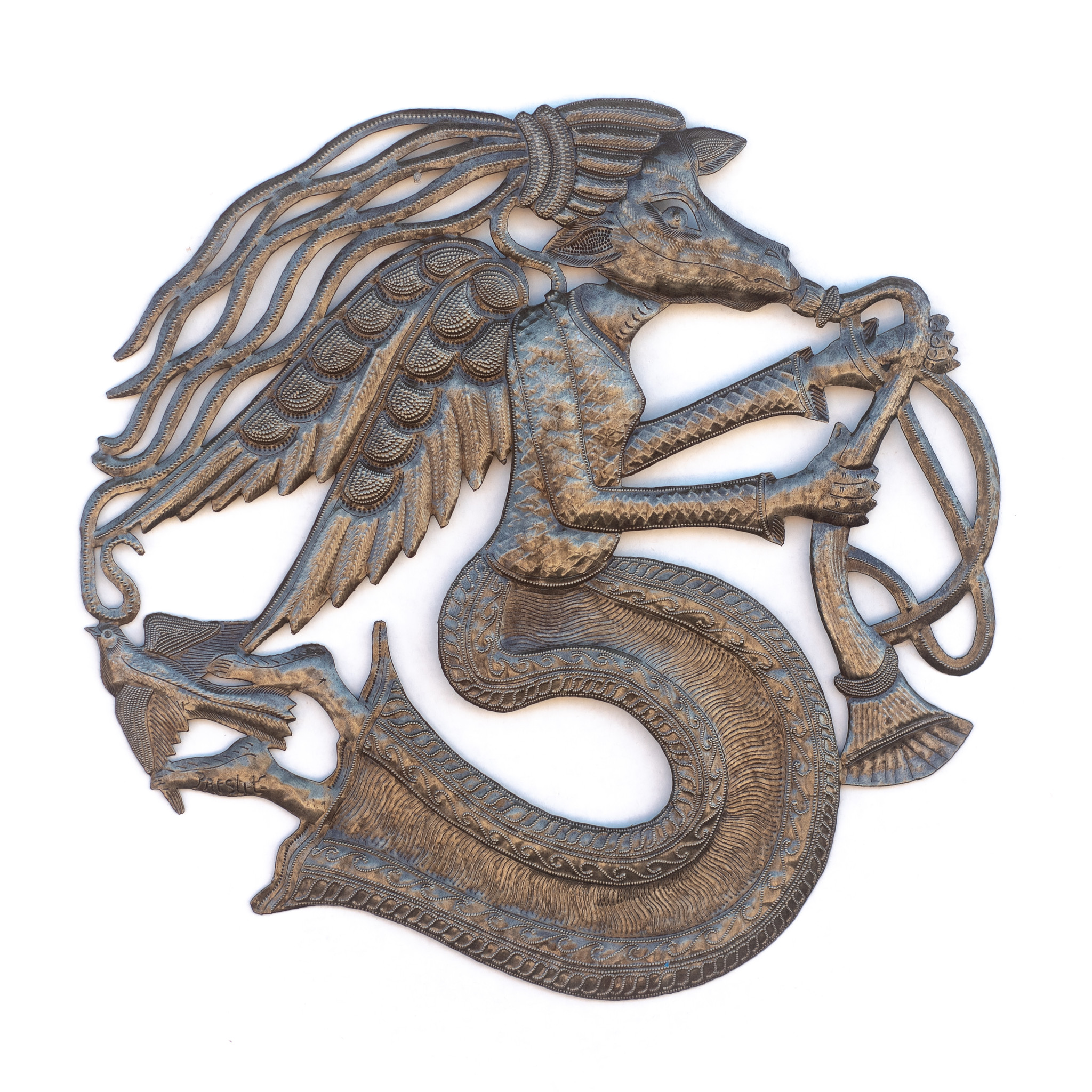The professionally photographed image depicts an intricate metal ornament featuring a fantastical hybrid creature with a cow's head and woman's body. The sculpture is predominantly tarnished silver with gold flecks and touches of blue and brown. The creature's legs curl unnaturally, poking out from beneath a skirt or robe, akin to a mermaid's tail. Its long hair, resembling dreadlocks or tied in a ponytail, transforms into branches. Angelic wings adorn its back, and it plays a brass instrument with an intricate S-shaped loop. Near its feet, a bird is sculptured, adding to the whimsical nature of the piece. The detail and craftsmanship suggest it is a unique, professionally made metal artwork.